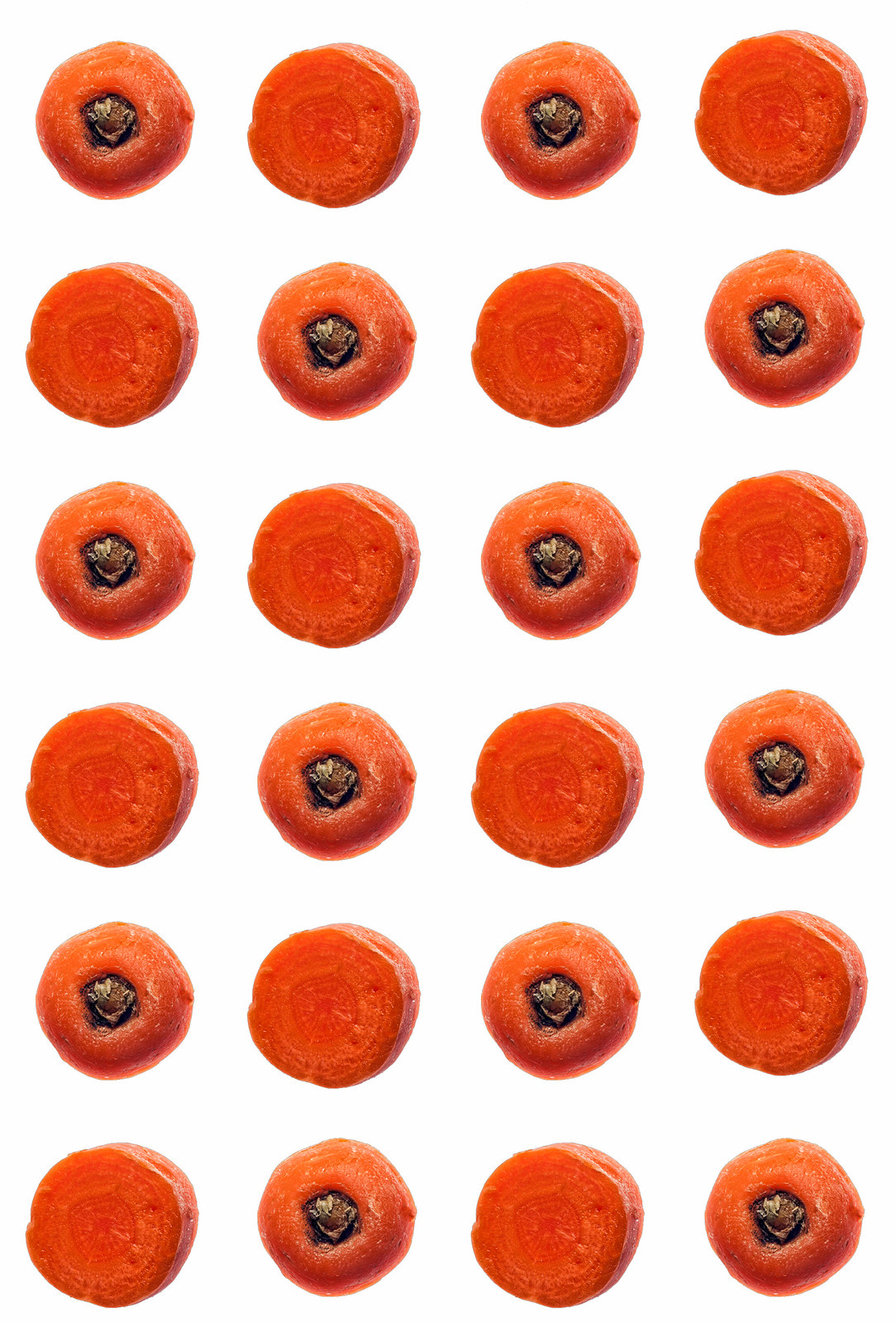This is a well-organized digital image showcasing 24 meticulously sliced carrot pieces arranged on a completely white background. The carrot pieces are laid out in six rows and four columns, alternating between top and interior slices. The top slices are distinguished by an orange exterior with a blackish-brown to gray stub where the stem was cut off, while the interior slices display a bright orange core with a lighter, sometimes yellowish, outer ring. The pattern repeats in an alternating fashion, starting each row with either a top slice or an interior slice, creating a visually symmetrical arrangement. The vivid orange of the carrot contrasts sharply with the pristine white of the background, highlighting the precise, circular cuts of each piece. Each carrot slice mirrors the others in shape and size, suggesting a digitally duplicated presentation for consistency and clarity.